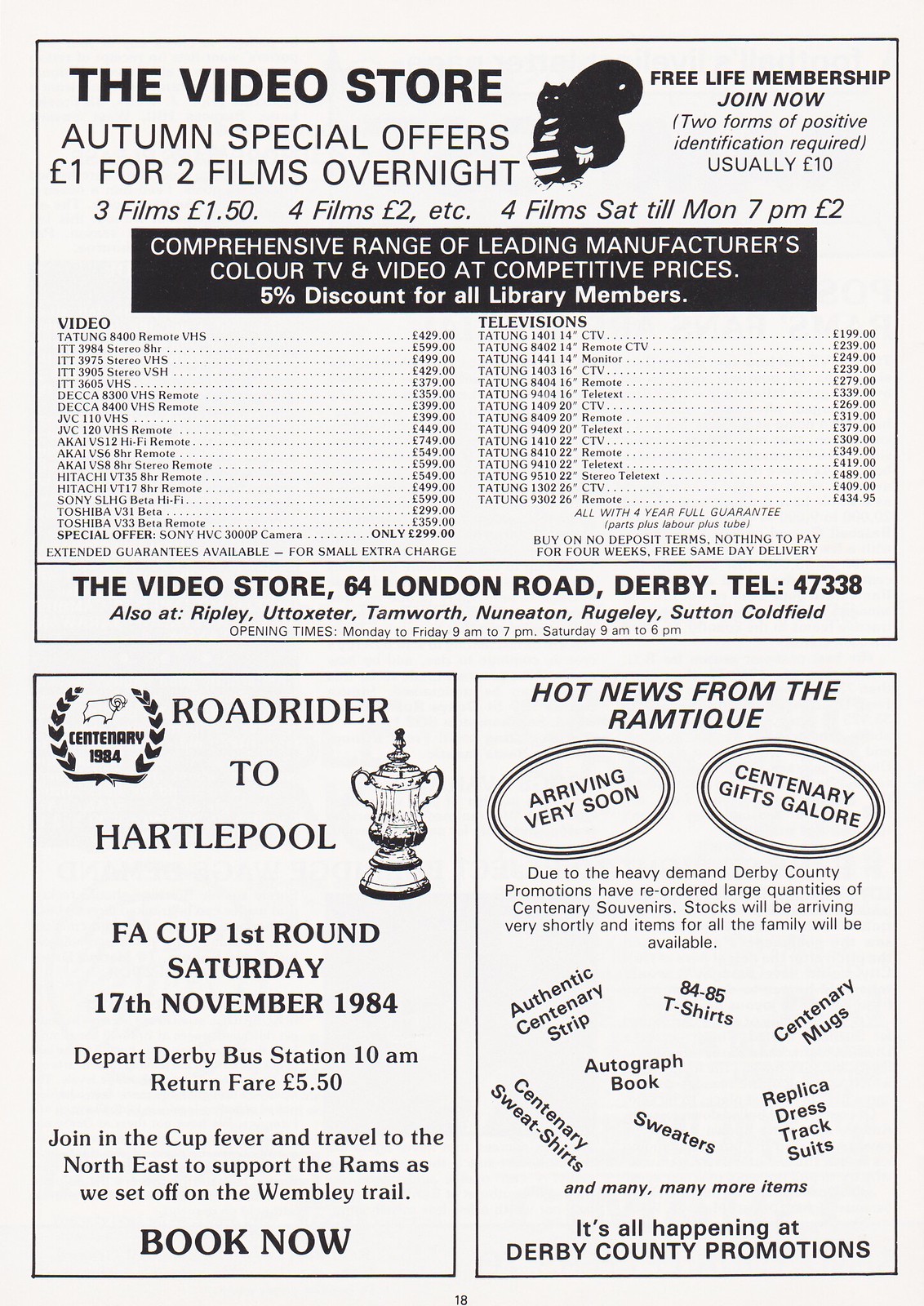This image depicts a printed flyer in black ink on white paper, featuring an advertisement from 1984. It is separated into three sections by a thin black border. The top half, labeled "The Video Store," is headlined in bold print and offers an "Autumn Special" of £1 for two films overnight along with a promise of free lifetime membership. This section also includes a black and white squirrel logo and provides the store's address and other locations. The lower half of the flyer is divided into two columns. The left column advertises a football event: "Road Rider to Hartlepool" for the FA Cup first round on Saturday, November 17, 1984, departing from Derby bus station at 10 a.m. with a return fare of £5.50. It encourages fans to join the Rams’ supporters traveling for the match. The right column announces hot news from "The Ram Teak," promoting Centenary gifts arriving soon. This section is part of Derby County Promotions. The entire layout captures various promotional offers and community events, firmly rooting it in its 1984 context.